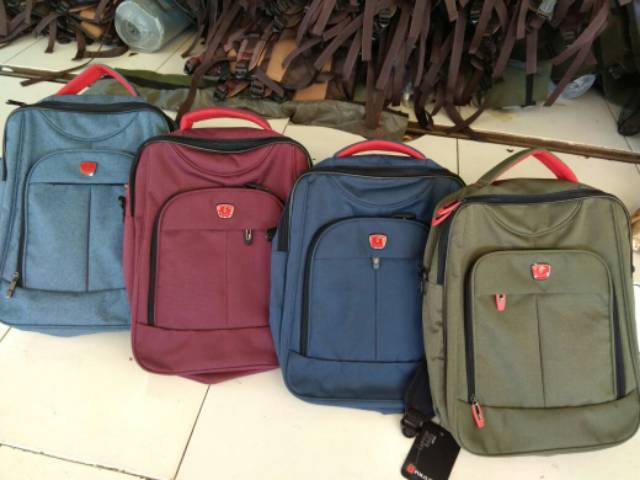The image depicts a white tiled floor with four book bags arranged diagonally on top of each other, allowing visibility of each bag. The bags are identical in style but vary in color: the bottom one is light blue, followed by a burgundy bag, then a navy blue bag, and finally an olive green one. The handles of each bag feature a reddish color inside, and they all have a reddish emblem. The book bags are adorned with black zipper pulls, except for the green one, which has orange zipper pulls and still carries the manufacturer's tag. In the background, there is a tiled step filled with various items, including what appears to be the bottom of a jug, a can, and a webbed material. The tile on both the floor and the step appear dirty within the crevices.